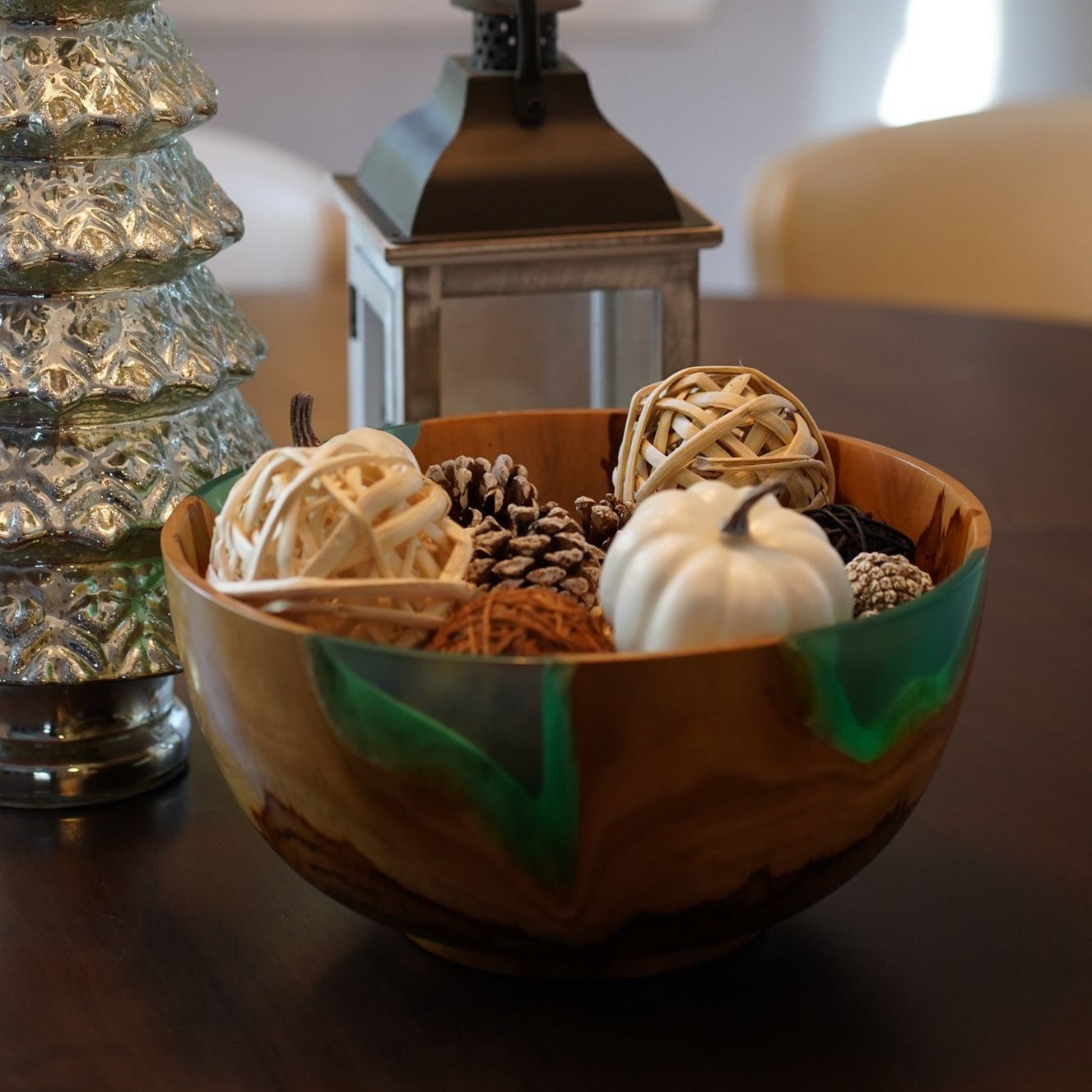In this color photograph, a close-up shot captures a wooden decorative bowl perched on a round cherry wood table. The bowl features dark wood grain at the bottom, transitioning to areas painted green near the top. Inside the bowl are several decorative items, including two wooden balls, multiple pinecones, and a small white pumpkin, which appears to be an art piece. The arrangement is complemented by a metal lantern with a black top and glass sides, positioned directly behind the bowl. To the left, a pewter-style figurine of a Christmas tree stands as an additional decorative element. In the blurred background, the tops of chairs are faintly visible, enhancing the cozy and detailed setting.